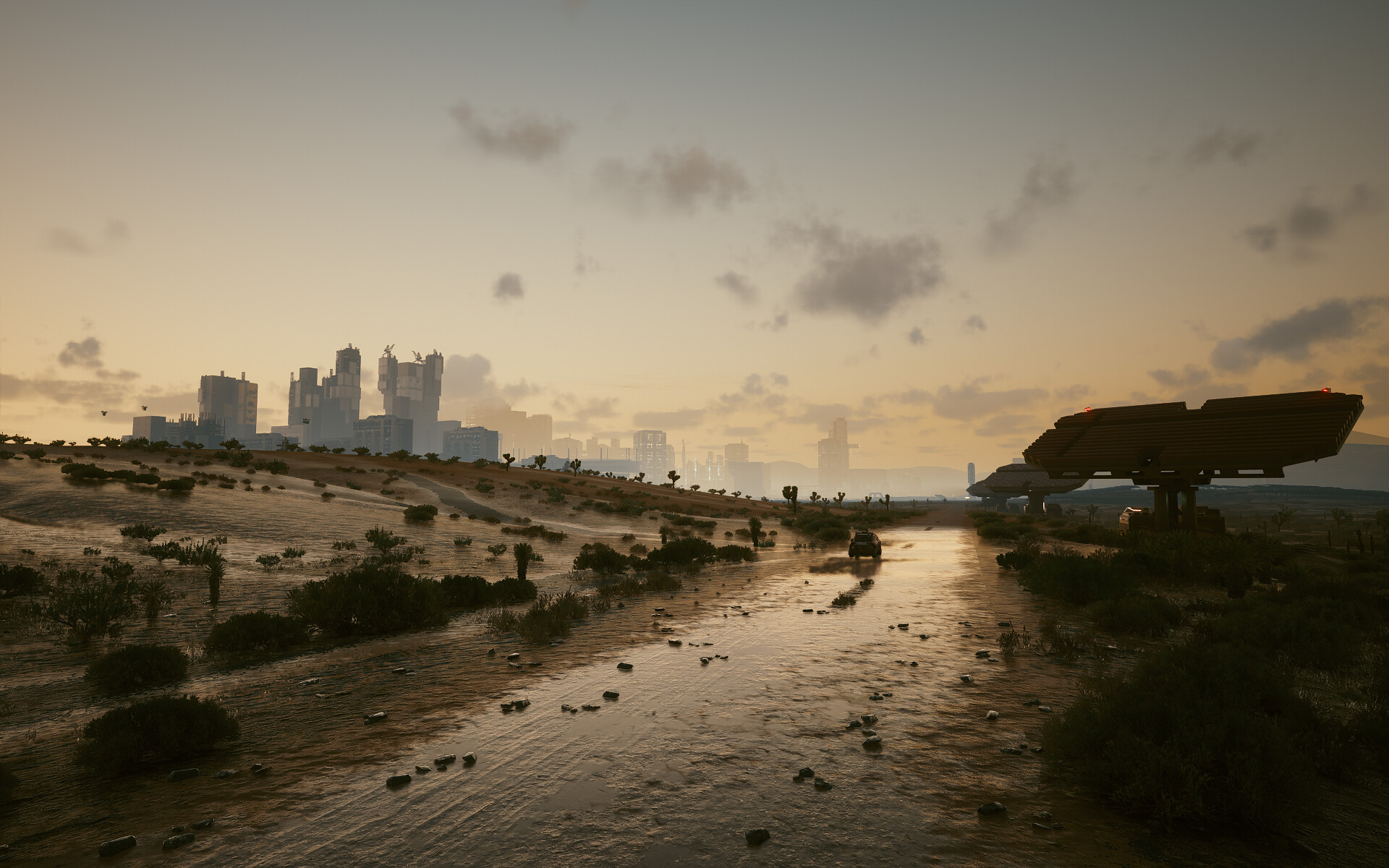A sepia-toned photograph captures a solitary car driving down an unpaved road, meandering through a barren desert landscape punctuated by sparse scrub brush. On the right side of the road, a large structure resembling a solar panel, mounted on a post, towers prominently with two conspicuous red lights affixed to it. In the hazy distance, the silhouettes of tall buildings emerge faintly, adding an element of depth to the scene amidst the pervasive dustiness. The sky above transitions subtly from scattered clouds to a gradient of brownish-orange hues near the horizon, evoking a sense of endless expanse and arid desolation.